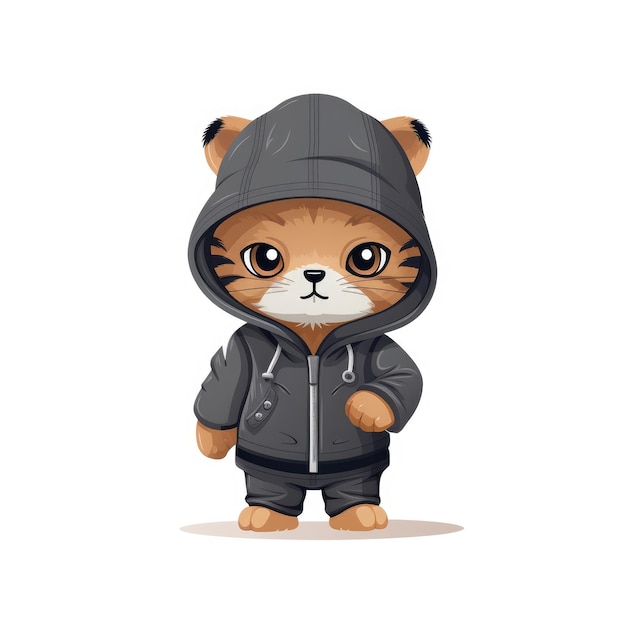This image is a digital illustration in a modern cartoon style of a personified cat resembling a baby tiger. The cat is standing upright on its back feet with a large, anime-style head and large brown eyes, gazing directly at the viewer. Its fur is light brown with black stripes on its cheeks and black tufts on the tips of its ears, giving it a cute and youthful appearance. The cat's white muzzle forms a triangular shape around its nose and mouth, complete with a small button nose and whiskers. 

It is dressed in a black hoodie and black pants, with the hood featuring holes for its rounded ears to poke through. The hoodie has strings and fits snugly around the cat's head and ears, emphasizing its adorable, childlike demeanor. The cat’s fur is depicted realistically, with detailed textures and shadow work that add depth to the illustration.

One of its hands is raised while the other rests by its side, and there is a light brown shadow beneath the figure, enhancing the sense of dimension. There is no background or text in the image, drawing full attention to the charming, anthropomorphic cat.